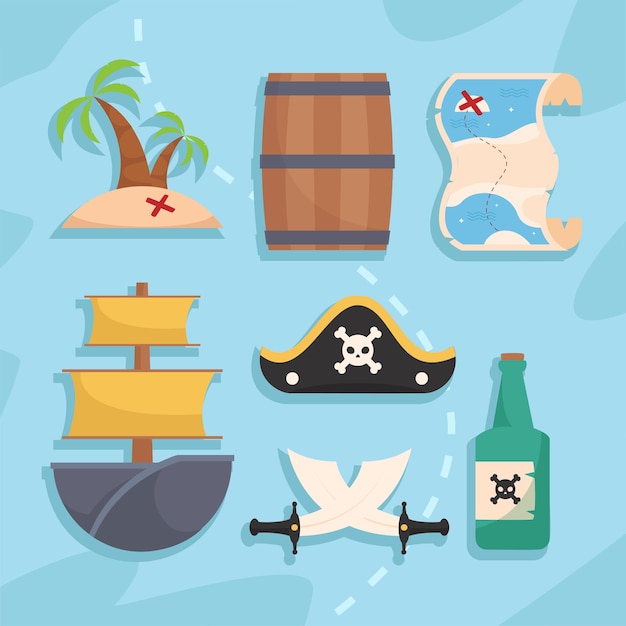This cartoon illustration features a pirate theme with a detailed array of pirate-related elements. The background mimics a sea with two shades of blue suggesting waves, and a swirling dashed line resembling a treasure map trajectory runs through it. Starting from the top left and moving clockwise, the illustration includes a palm tree icon with a red X below it, signifying a treasure spot, positioned on a small sandy mound. Adjacent to the palm tree is a wooden barrel, followed by a treasure map showing another red X at the top left corner. Next is a sea-green bottle with a cork, displaying a skull and crossbones design on a white label, symbolizing poison or pirate grog. Continuing around, there are two crossed pirate swords with black handles. A detailed pirate ship with gray sails and hull appears next, followed by a central black pirate hat featuring a yellow border and a prominent white skull and crossbones symbol flanked by two white dots on either side. The illustration is completed with light and beige tones on the map and intricate details, making it a vivid collection of pirate imagery.